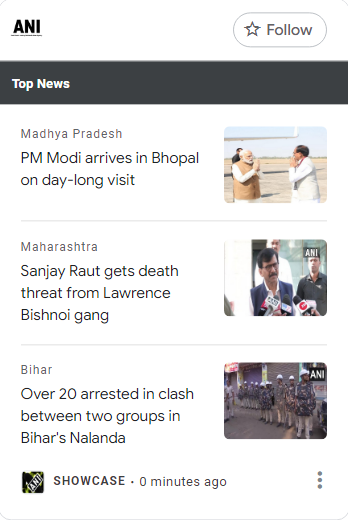**Image Caption:**

At the top of the image, the background is white with the black text "A and I" on the left-hand side. To the right, there is a gray-outlined star with the word "follow" written in gray inside it. Below this, there is a section with a dark gray background. The text "Top Notes" is written in white.

Underneath "Top Notes", in black text, it reads: "MADHYA PRADESH PMOD arrives in BHOPAL on day-long visit." A thin gray line separates this section from the rest.

Following the gray line, the text "MAHARASHTRA" appears in gray. Below it, in black text, it says: "Saundry RAUT gives death threats from Lawrence BISHNOI gang." Another thin gray line runs across the image.

Next, the text "BIHAR" is in gray, followed by the black text: "Over 20 arrested in clash between two groups in BIHAR'S NALANDA."

At the bottom of the image, there is a black square box with "A and I" in white capital letters inside. Next to this box, in black capital letters, it says "SHOWCASE." Additionally, there is a small black circle indicating "0 minutes ago."